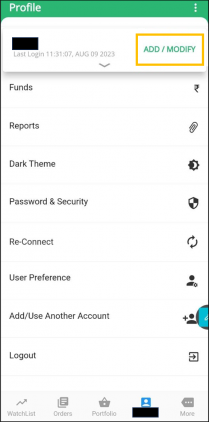The image depicts a vertically oriented rectangular interface, bordered by a thin black line. At the top, a green strip spans the width of the rectangle, with the word "Profile" in white text on the left side and three vertically aligned white dots on the right side. Below this, on a white background, there is a section obscured by a black rectangle, beneath which it reads "Last logged in 11-31-07 August 9, 2023."

To the right, green text reads "Add Money" and "Modify," encapsulated within a yellow box. Further down, left-justified links are listed as follows: "Funds," "Reports," "Dark Theme," "Passwords and Security," "Reconnect," "User Preference," "Add Use Another Account," and "Log Out." 

At the bottom, navigation options including "Watch Lists," "Orders," "Portfolio," and "Profile" are presented; however, the profile name is blocked out by a black rectangle. The link "Add Use Another Account" is accompanied by a bubble and a green box, the function of which is unclear. The color palette of the interface includes black, white, green, gray, yellow, blue, and turquoise, with faint gray lines separating each item on the white background.